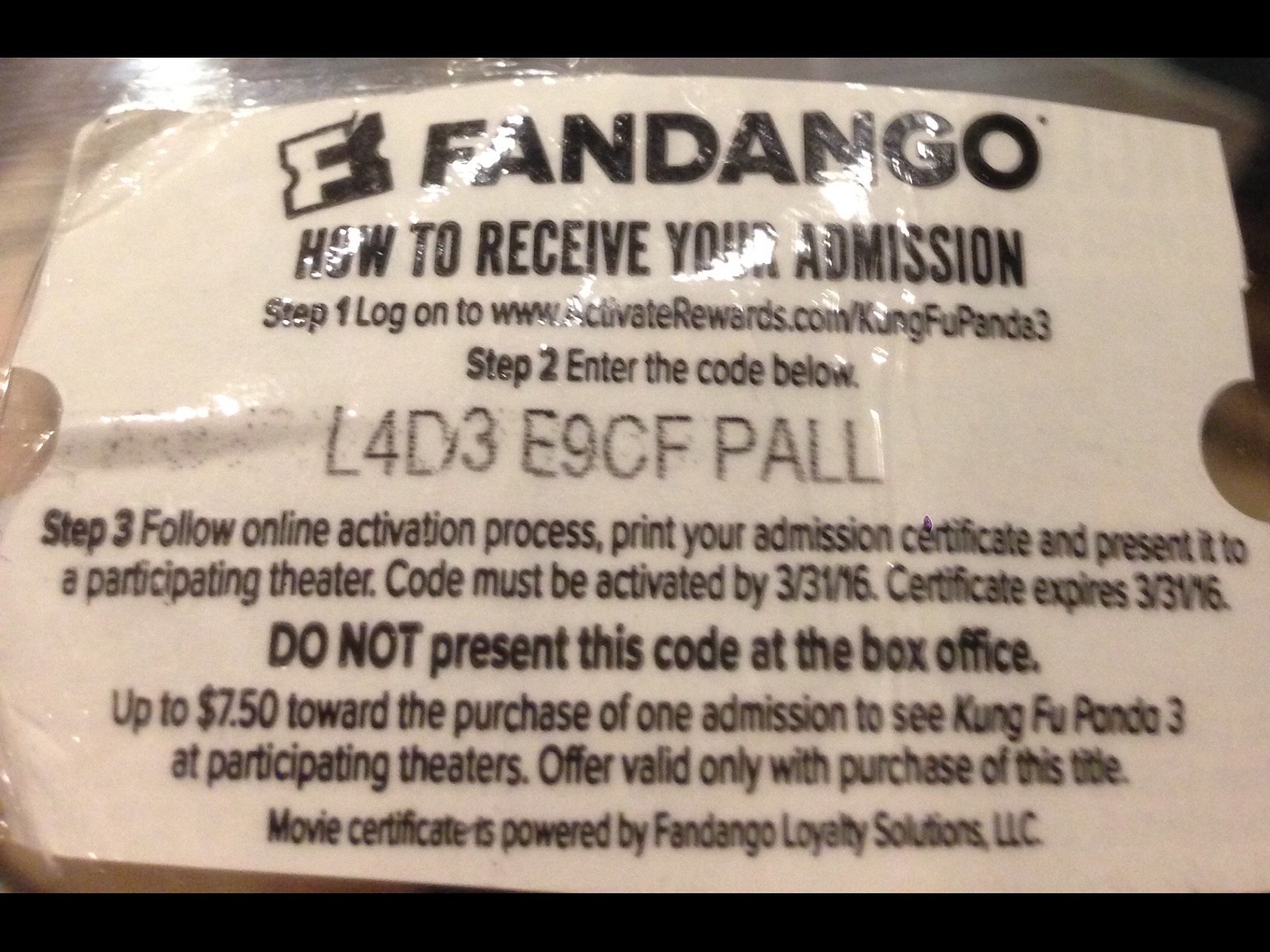A photograph of an off-white sticker, slightly tilted. The header prominently displays "Fandango" in bold, followed by smaller text detailing the instructions for redeeming a movie ticket for "Kung Fu Panda 3." Step 1 directs users to log on to www.activaterewards.com/KungFuPanda3. Step 2 instructs them to enter the provided code. Step 3 explains the process of following the online activation instructions, printing the admission certificate, and presenting it at a participating theater. The sticker also notes that the code must be activated by March 31, 2016, and the certificate expires on the same date. A final caution advises users not to present the code directly at the box office.